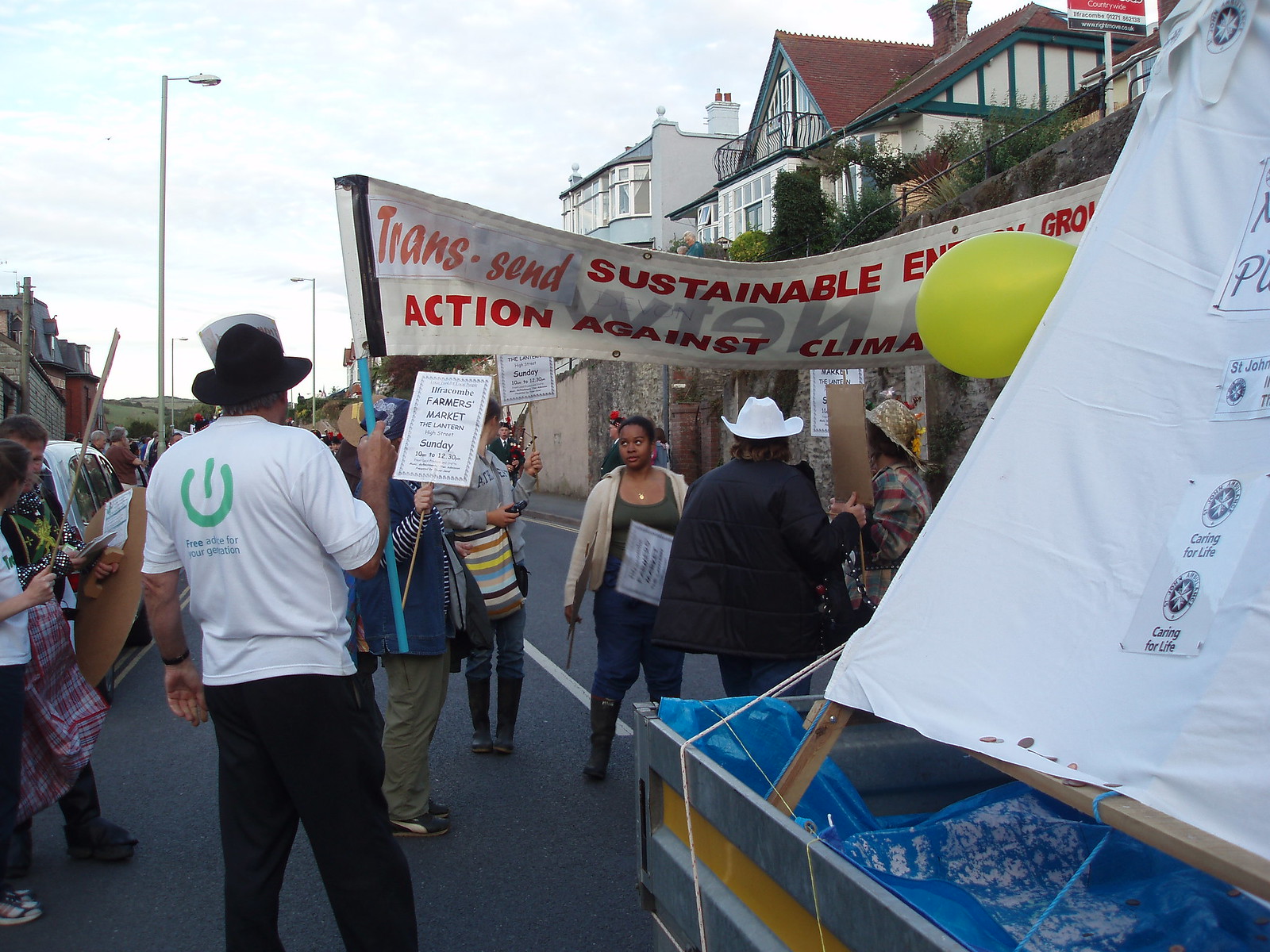In the center of the image, a group of protesters march on an asphalt road during the middle of the day, holding a large white banner with red text that reads, "Transcend Sustainable Energy Action Against Climate Change." The scene is set against a cloudy sky, and various signs can be seen among the crowd, including ones that read "Haricom Farmers Market," "The Lantern," and "High Street, Sunday 10 p.m. to 12:30 p.m." To the right, a couple of buildings frame the street, while in the bottom right corner, there is a cart with a sign on it, possibly part of the protest or an adjacent market. The color palette of the image includes blue, white, yellow, green, black, different shades of blue, and brown, reflecting the diverse elements within the scene. The overall setting is an outdoor climate protest with a clear focus on sustainable energy and action against climate change.